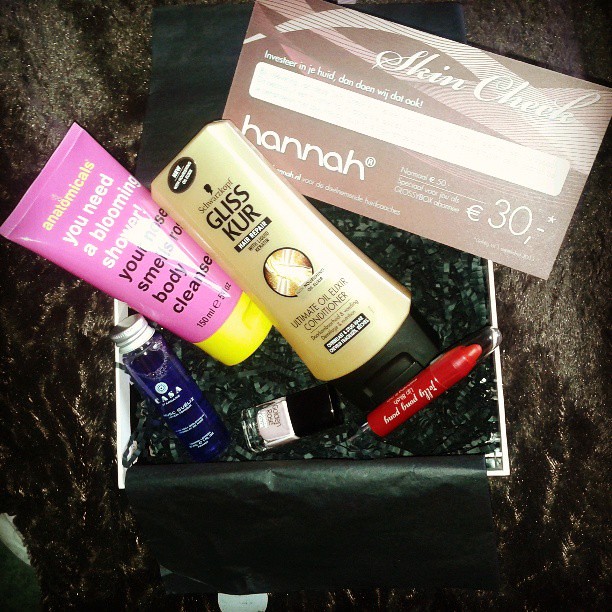This photograph showcases a meticulously arranged gift basket filled with a range of toiletry and cosmetic products, nestled in a decorative metal basket lined with green crinkled paper. Among the prominent items, there is a pink lotion tube that reads "Anatomicals - You Need a Blooming Shower, Your Nose Smells Rose Body Cleanser." Another significant item is a golden bottle labeled "GLISS KUR Ultimate Oil Elixir Conditioner." In addition, there's a blue liquid bottle with a silver cap and a small white nail polish bottle branded "Golden Rose" with a black cap. A striking feature is the dark, rock-like marble table surface beneath, glistening with embedded sparkles and crystals. Various other beauty tools, including a makeup application stick and potentially more nail care items, add to the assortment, making this basket a comprehensive beauty care collection. The larger items such as the lotion and conditioner align from the upper left-hand corner to the lower right, while the smaller nail care items are arranged from the lower left to the upper right, creating a visually appealing display.